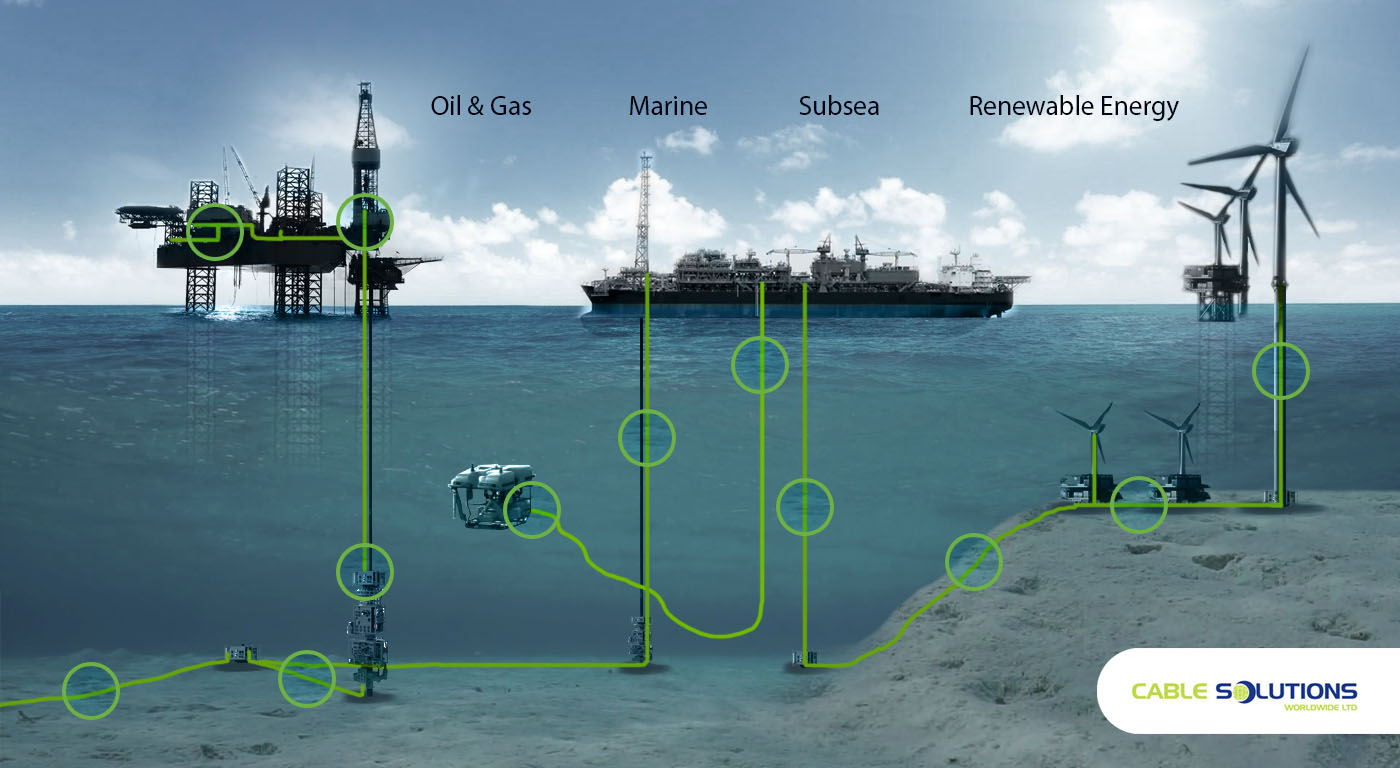This advertisement for Cable Solutions features a detailed diagram illustrating the interconnectedness of oil and gas, marine, subsea, and renewable energy sectors. Starting at the bottom, the beach leads into the ocean, where various key components are positioned. To the left, there is an oil and gas rig, followed by a giant oil tanker in the center. On the right side stands a tall, ambiguous tower-like structure. Beneath these elements floats a large block on the water's surface. The foreground of the image includes wind turbines positioned along the beach at the bottom right. Green circles highlight various points of interest, including the ships and along the beach, which are interconnected by lines, demonstrating how Cable Solutions’ products integrate with these different industries. The top of the image prominently features the words "Oil and Gas, Marine, Subsea, and Renewable Energy," while the company name, Cable Solutions, is marked in the bottom right corner. The image captures both the water and seabed below, with clouds visible on the horizon, emphasizing the comprehensive scope of the company’s capabilities across different environments.